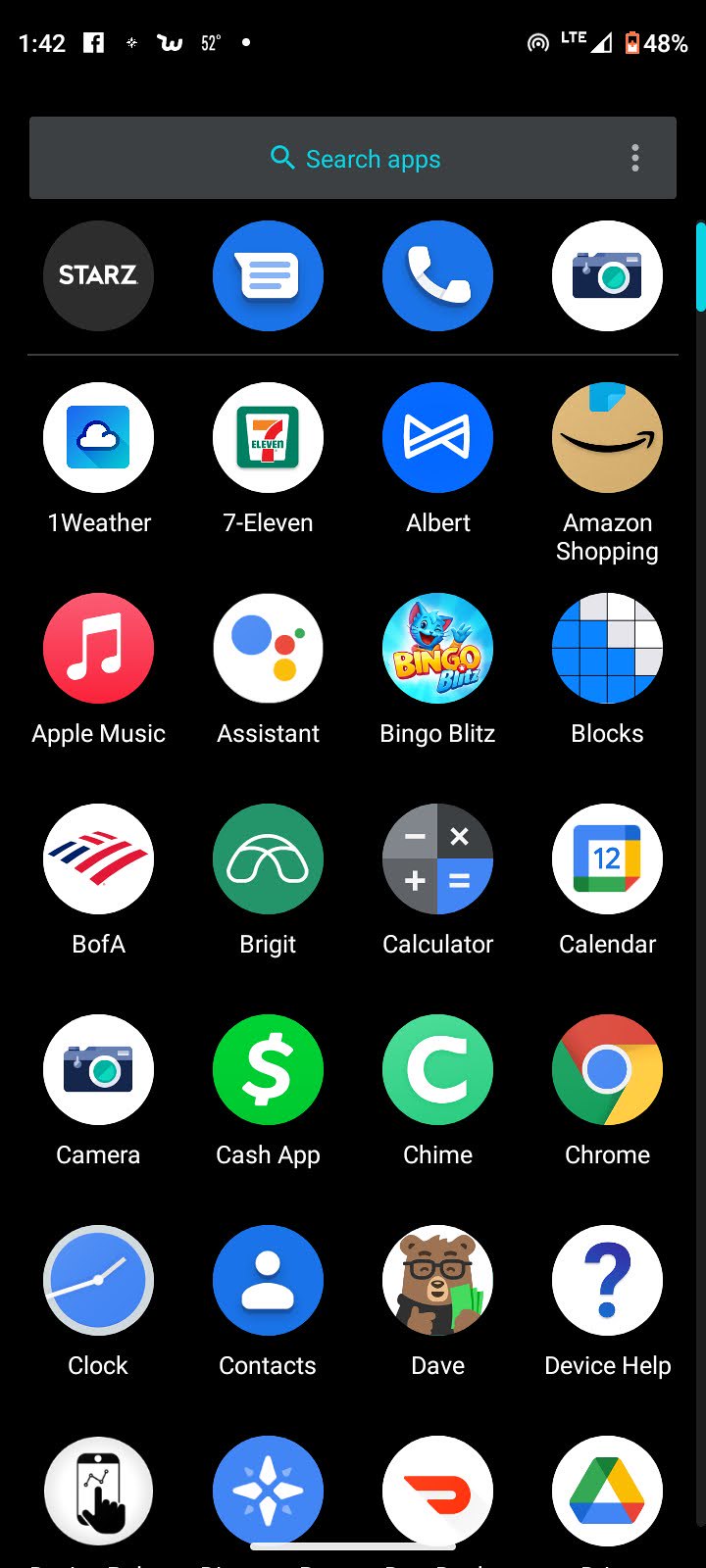This image is a screenshot of a cell phone screen with a completely black background. At the top of the screen, there is a search bar displaying "Search apps" in blue accompanied by a magnifying glass icon. There are 28 application icons arranged in a grid layout, all with blue-themed logos. 

From left to right, top to bottom, the application icons are as follows:

1. **Starz** - Streaming service logo.
2. **Messenger** - Chat application logo.
3. **Blue Circle with a White Telephone** - Possibly a calling or contact app.
4. **White Circle, Blue Box** - Unidentified application with a blue box inside a white circle.
5. **The Cloud** - Cloud storage or service app.
6. **1Weather** - Weather forecasting app.
7. **7-Eleven** - Convenience store app featuring the 7-Eleven logo.
8. **Albert** - Financial app with a blue logo and almost triangular affinity sign.
9. **Amazon Shopping** - Online shopping app featuring the Amazon logo.
10. **Apple Music** - Music streaming service.
11. **Assistant** - Likely Google Assistant with a circular icon.
12. **Bingo Blitz** - Game app featuring bingo.
13. **Blocks** - Possibly a game featuring blocks.
14. **Bank of America** - Banking application.
15. **Bridget** - Unidentified app, potentially financial or service-related.
16. **Calculator** - Standard mathematical calculator app.
17. **Calendar** - Calendar scheduling app.
18. **Camera** - Photo-taking application.
19. **Cash App** - Financial/transaction application.
20. **Chime** - Banking app.
21. **Chrome** - Google Chrome web browser.
22. **Clock** - Timekeeping app featuring alarm and stopwatch functions.
23. **Contacts** - Address book for storing contact information.
24. **Dave** - Financial app featuring a cartoon bear with glasses holding a green object.
25. **Device Help** - Assistance app for device troubleshooting.
26. **An icon of a black hand pointing at a graph on a cell phone** - Likely an analytics or tracking app.
27. **Blue Circle with White Four-Pointed Star** - Unidentified app; possible service or utility.
28. **DoorDash** - Food delivery service logo with a white background and blue circle.

At the very bottom, there are four additional applications:

1. **Google Drive** - Cloud storage with the Drive logo.
2. **An unidentified white icon against a black hand pointing at a graph on a cell phone** - Presumably, an analytics or performance monitoring tool.
3. **Blue Circle with White Four-Pointed Star** - Appears to be a service or utility application.
4. **DoorDash** - Food delivery application with a white background and blue circular logo.

Overall, this succinct layout of applications provides a broad mix of communication, financial services, entertainment, utility, and productivity tools, dominated by a blue color scheme.